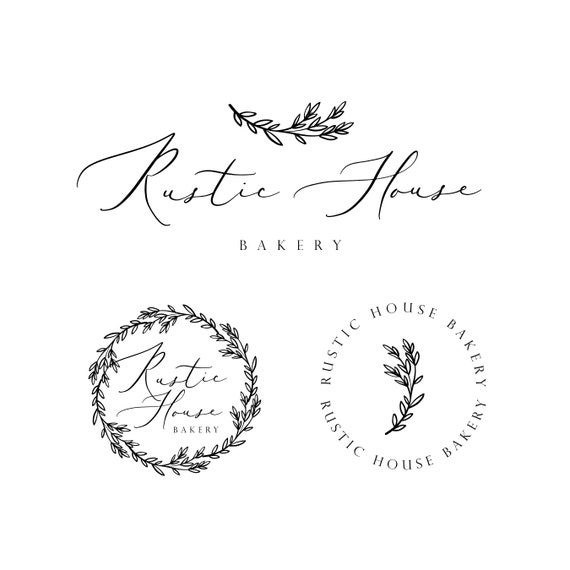The vertical image features a series of three different black and white logos for Rustic House Bakery, displayed without any outside border. At the top of the image, "Rustic House" is elegantly written in a very fancy, horizontal cursive style, with the word "bakery" printed below it in a more standard, possibly Times New Roman or Arial font. Above "Rustic House" lies a decorative branch, potentially of olive or wheat, adorned with leaves. 

Beneath this main logo, two circular logos are presented side by side. The logo on the left encircles the words "Rustic House" in cursive with "bakery" in block text, enclosed within a wreath-like border of the same leafy branch. The logo on the right mirrors this motif, with "Rustic House Bakery" written along the perimeter of the circle, both at the top and bottom, around a central figure of the leafy branch. These designs illustrate various conceptual approaches to the bakery’s branding, each incorporating consistent natural and elegant elements.